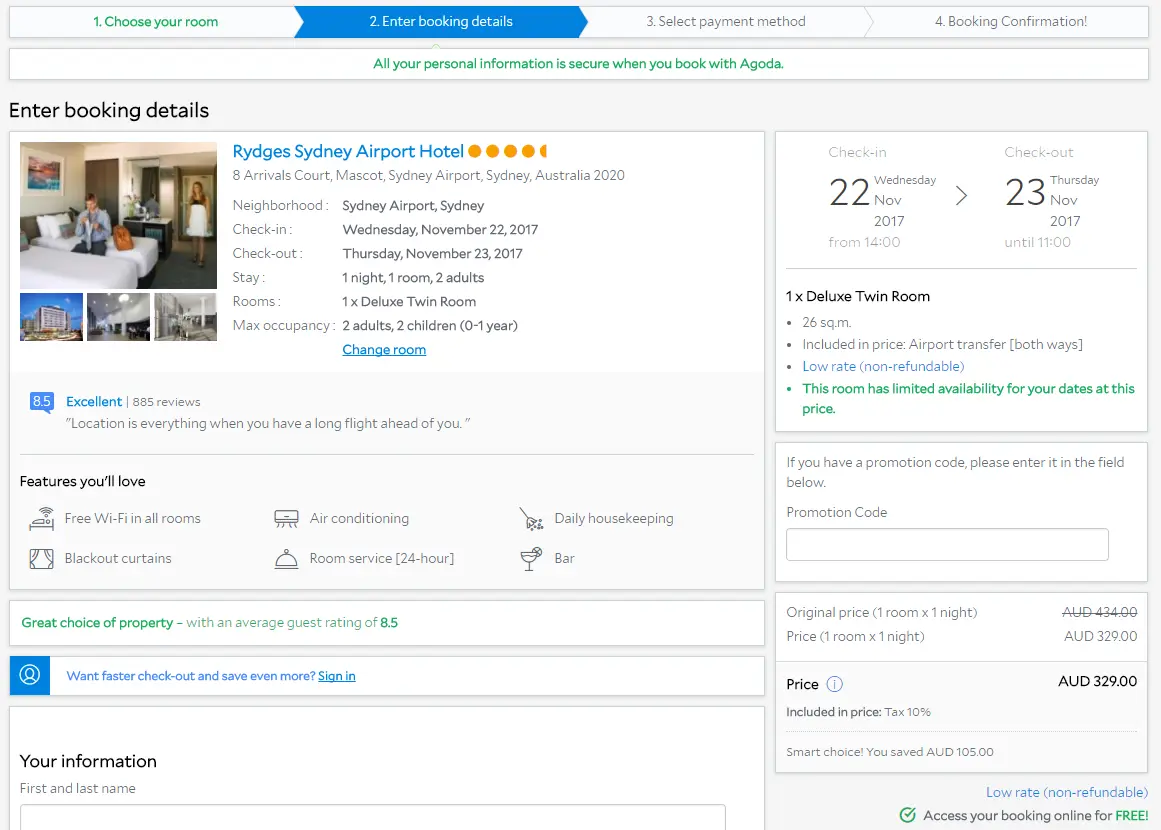Here is a detailed and cleaned-up caption for the described image:

---

The image is a screenshot from the booking process on Agoda's website, identified by the branding on the first two bars at the top of the page. The booking process is presented as a four-step system at the top: 1. Choose Your Room, 2. Enter Booking Details, 3. Select Payment Method, and 4. Booking Confirmation. The current step, "Enter Booking Details," is highlighted in blue with white text, while "Choose Your Room" appears in white with green text, and the subsequent steps, "Select Payment Method" and "Booking Confirmation," are grayed out with white backgrounds and gray text to indicate that they are upcoming steps.

Beneath the highlighted step, a tooltip reassures users that their personal information is secure when booking with Agoda. Below this, there is a field for entering booking details. The left-hand side of the screen shows details about the selected hotel: Bridges Sydney Airport Hotel, which has a quality rating displayed as four out of five orange circles. The hotel's location is listed as 8 Arrivals Court, Mascot, Sydney Airport, Sydney, Australia, 2020. The check-in and check-out dates are Wednesday, November 22nd, 2017, and Thursday, November 23rd, 2017, respectively. This information is mirrored on the right-hand side in a box that also displays the selected room type, a Deluxe Twin Room.

Additional information on the left includes a tooltip with reviews and features you'll love, along with average guest ratings. On the right-hand side, a small box highlights the room price, which is AUD 329. At the bottom of the image, there is a section to enter the first and last name, marking the initial entry point for the user's personal information.

---